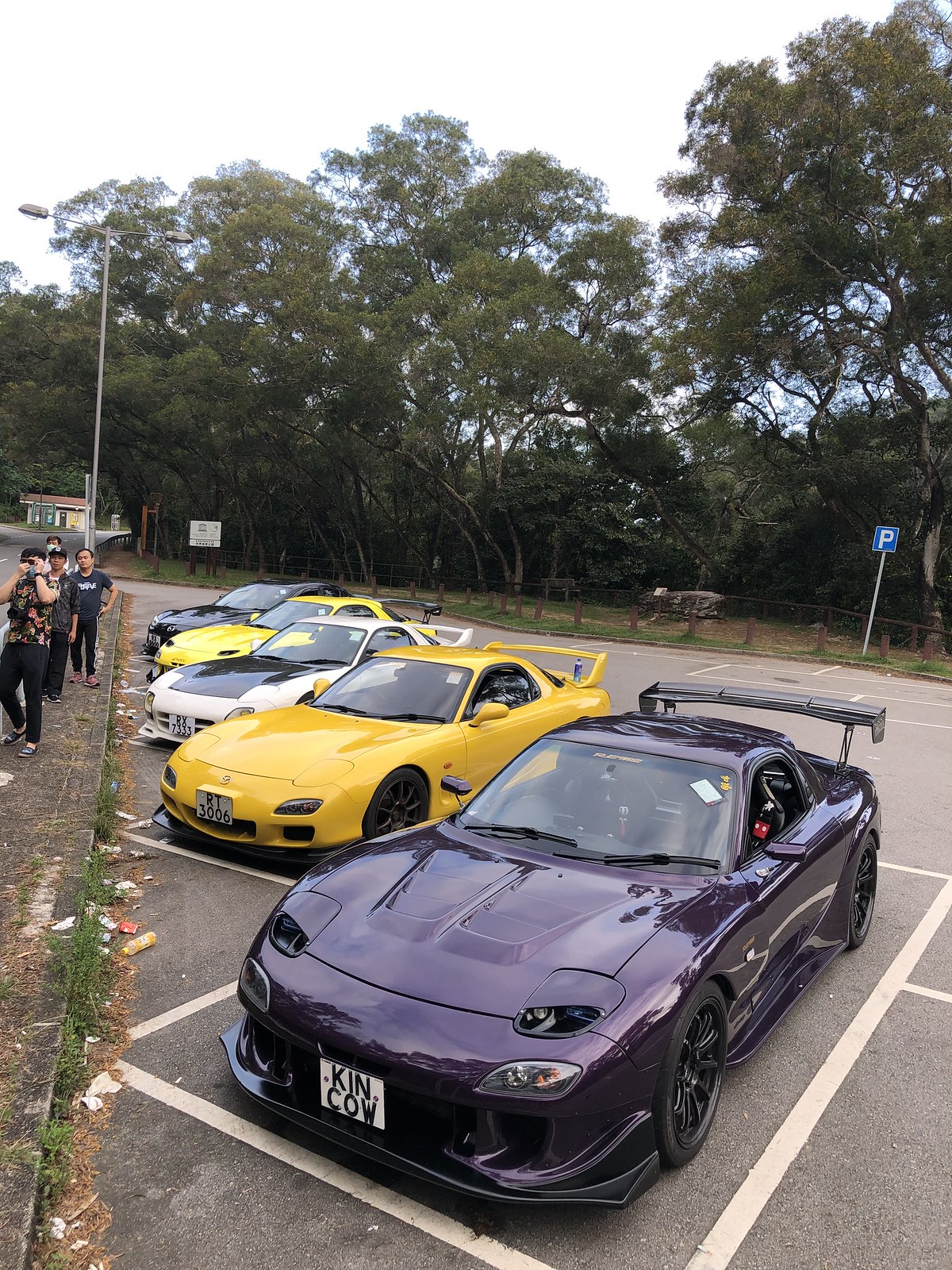In this outdoor photo, a gathering of five highly customized Mazda RX-7 sports cars is showcased. The cars, which include a black, two yellow, one white, and one striking midnight purple RX-7 with a unique license plate reading "K-I-N-C-O-W," are meticulously parked in angled spaces within a lined parking lot. The purple RX-7 stands out with its aggressive hood scoops, black bottom front bumper, and prominent aftermarket rear spoiler. A cloudy sky forms the backdrop, contrasting with the vibrant car colors. 

In the background, several people are observed walking along a pathway; one individual is taking a photo of the photographer. This scene is set against a backdrop of trees and distant buildings, with a parking sign visible on the right. The overall ambiance suggests a car meet or enthusiast gathering, with the cars arranged in a visually engaging manner and several onlookers possibly admiring their rides.